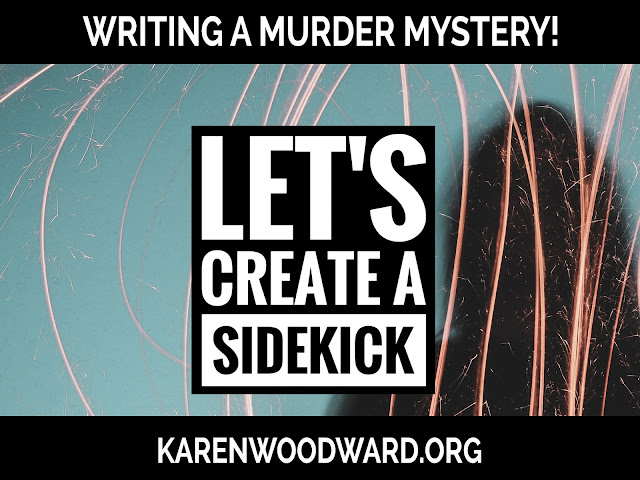In this digital graphic advertisement, we see a poster-like design with a rectangular shape. The background is predominantly a teal blue, accented with abstract light streaks and sparking embers, reminiscent of light trails from a time-elapsed photograph. These dynamic scribbles, in shades of gold and pink, add a sense of movement and energy to the image.

The layout includes prominent black bars at the top and bottom of the image. At the top, in all capitalized white text, it reads "WRITING A MURDER MYSTERY!" This bold announcement establishes the theme of the graphic.

Central to the design is a large black box containing the white text "LET'S CREATE A SIDEKICK." The word "sidekick" is further emphasized in black text against a white rectangle, making it stand out prominently.

On the lower right, a black shadowy silhouette of a woman’s head and shoulders adds a mysterious and human touch to the graphic. The bottom black bar, or footer, in all caps white text, features the website "KARENWOODWARD.ORG."

The cohesive use of color and text positions, combined with the abstract yet striking background, make this a compelling and eye-catching digital advertisement.